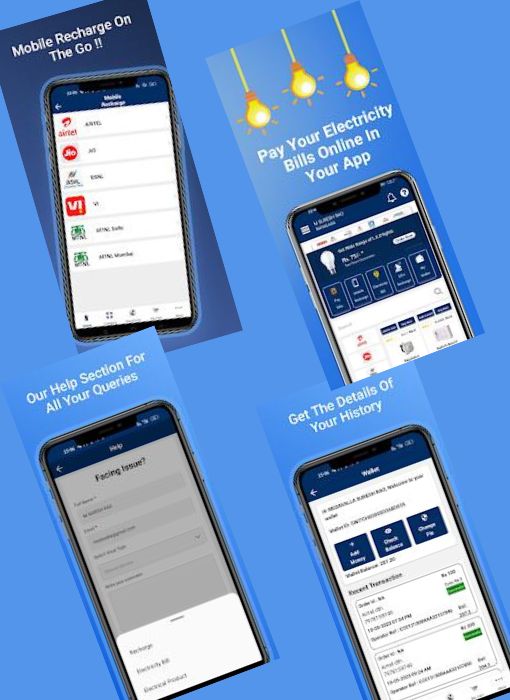A promotional image for a mobile app is set against a blue background. The image features four angled screenshots of a cell phone, each with its own specific background and label, detailing the app's various functionalities.

1. **Top Left**: Titled "Mobile Recharge on the Go," this section showcases a white screen filled with red and green icons arranged in six rows. These icons likely represent various features or options available within the app. The background for this section is a darker shade of blue.

2. **Top Right**: "Pay Your Electricity Bills Online" is highlighted here. It features a blue background with three hanging yellow light bulbs. The phone's screen displays a small window containing text and options, though the details are too tiny to decipher clearly.

3. **Bottom Left**: This portion, labeled "Our Help Section for All Your Queries," displays a gray background with faint text that appears to read "Facing Issue?" This suggests it is meant to assist users with troubleshooting and support.

4. **Bottom Right**: Under the heading "Get the Details of Your History," we see a clear blue background with slightly blurred white text at the top, possibly saying "Wallet." This section includes three horizontal dark blue squares followed by two white windows containing information, each accompanied by a rectangular green button on the right.

Overall, this advertisement visually communicates the app's key features such as mobile recharge, bill payments, support section, and transaction history, designed to enhance user convenience.